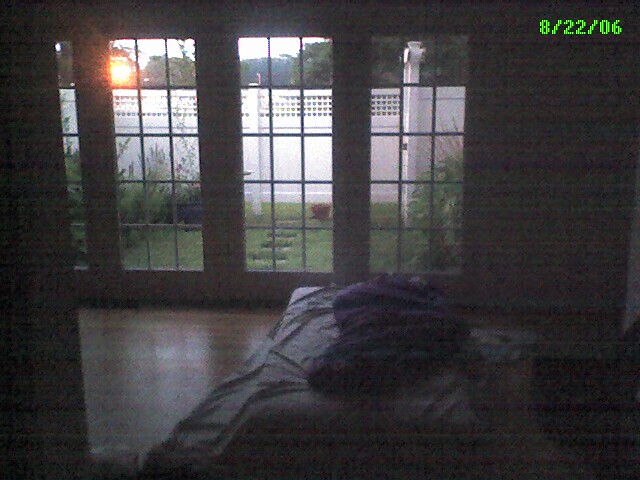In the top right corner of the image, a green timestamp reads "8-22-06." On the far right side, there is a mattress on the floor, covered with a bunch of folded, wrinkled blankets and a bedsheet spread messily around. A person seems to be lying on the mattress, wrapped in a sleeping bag. In the background, there are doors with window panes arranged in a 3 by 5 grid, with the height being taller. Through the window panes, a view of a lawn with grass and a white wooden fence is visible. Sunlight streams through the top left corner, illuminating green tree leaves at the top back and some grass growing at the bottom.